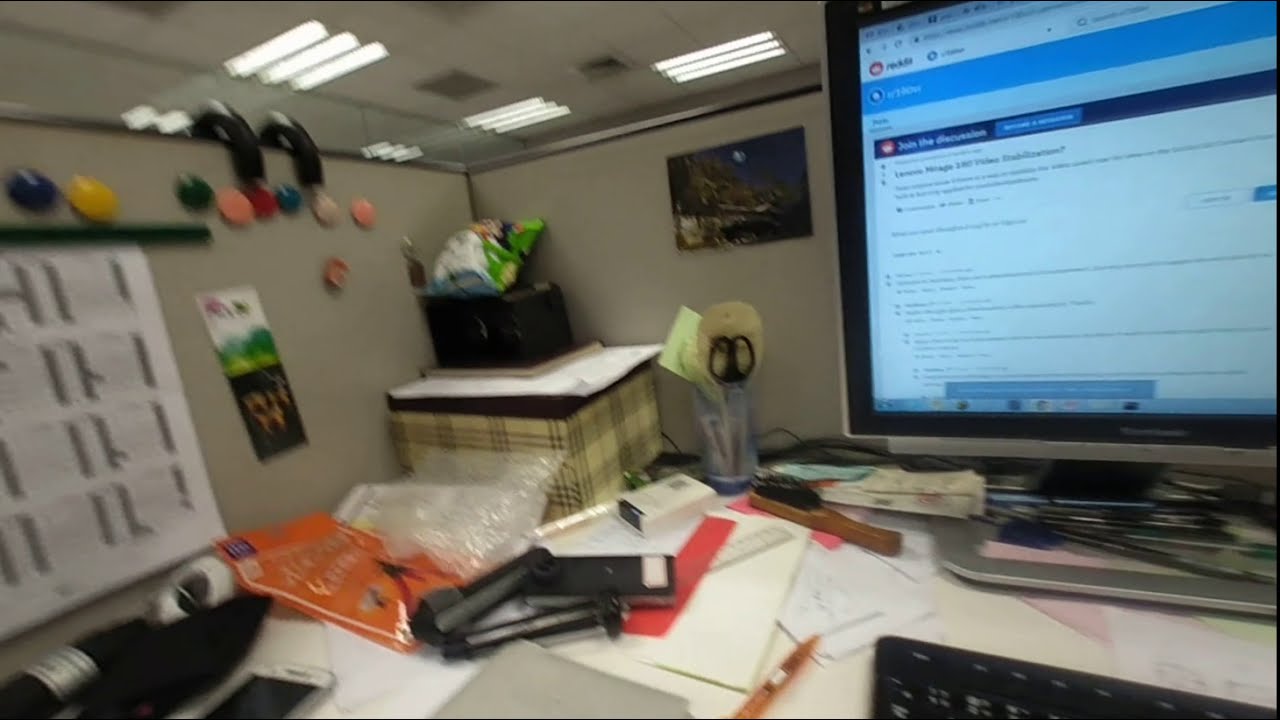This image captures a cluttered office cubicle with a computer monitor displaying Reddit, suggesting it might be a screen capture from a video due to its slight blur. Dominating the scene, the computer monitor sits to the right, while the tip of a black keyboard is barely visible. The cubicle walls are off-white, and the left wall features a calendar or planner alongside various colorful pushpins—blue, yellow, green, pink, red, teal, tan, and pink. The corner of the cubicle holds a plaid yellow container with another box on top, and a bag of chips rests within this setup. Scattered across the messy desk are envelopes, papers, wrappers, and packing materials. Typical office supplies, including a glass holding pens and scissors, can be seen. The overhead white-tiled ceiling is equipped with embedded fluorescent lights, vents, and speakers, contributing to the typical office ambiance.